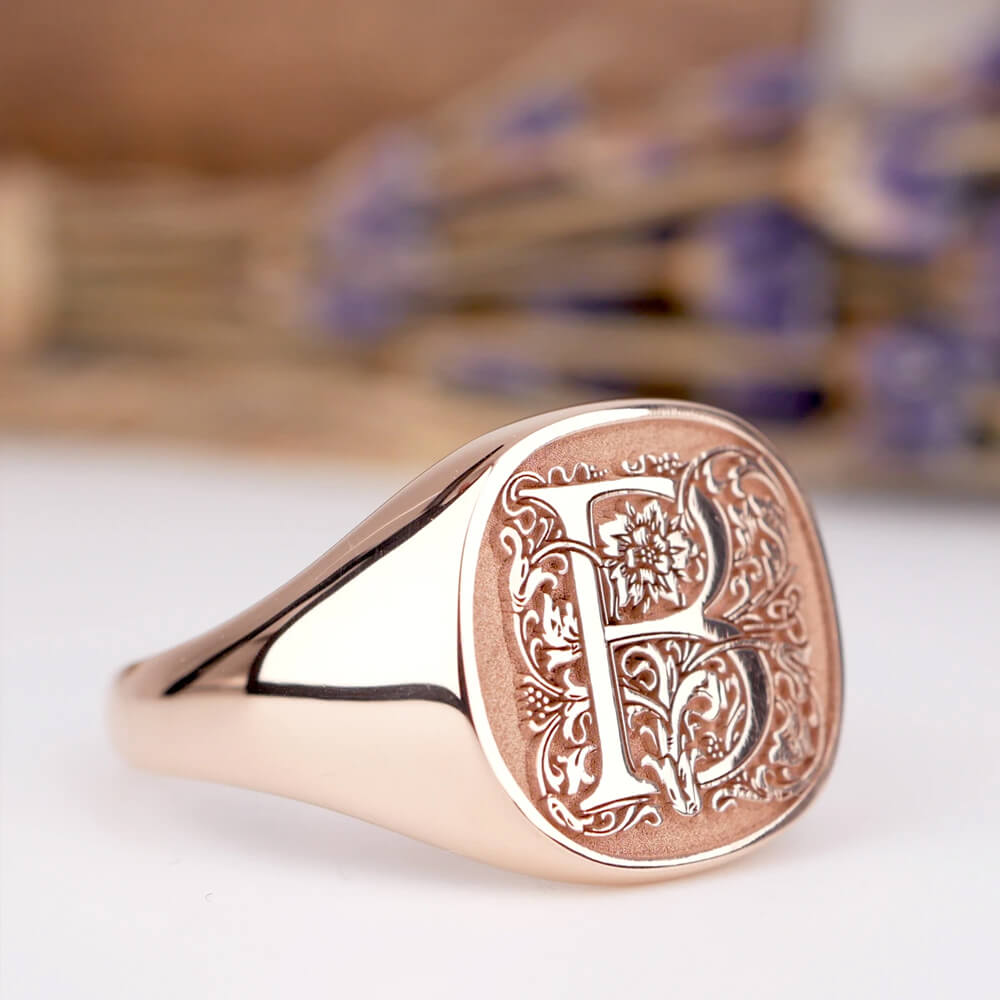The photograph captures a close-up of a finely crafted ring positioned on a clean, white surface. The ring itself is made of a unique peach-colored metal with intricate decorative designs. At its center, a prominent capital "B" is engraved, surrounded by twirling vines and a flower blossom embedded at the top of the letter. The ring exudes elegance and appears to be of significant value, likely designed for a man's wear. The background is blurred, showcasing an indoor setting with natural lighting, revealing a mix of brown and hints of blue colors, adding an enigmatic ambiance to the otherwise detailed focal point. Farther back in the distance, there's a subtle hint of something purple, though it remains undefined and out of focus, enhancing the mystery of the scene.